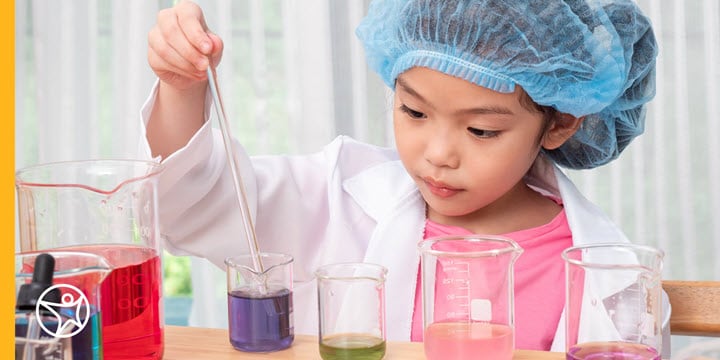The photograph captures an indoor scene featuring a young, light-skinned Asian girl engaged in a science experiment. She is dressed in a pink t-shirt layered under a white lab coat and wears a blue hairnet to keep her hair tidy. In the foreground, a light brown table extends from the left and continues off-screen to the right, topped with various glass beakers and jars containing brightly colored liquids, including red, purple, green, and pink. Detailed markings on the containers indicate their measurements. The girl, seen from the chest up, has her right hand raised, holding a long glass pipette which she uses to stir one of the beakers filled with purple liquid. Behind her, partially transparent white curtains form the background, enhancing the indoor setting's soft lighting. The image is framed by a dark yellow border that adds contrast to the scene.